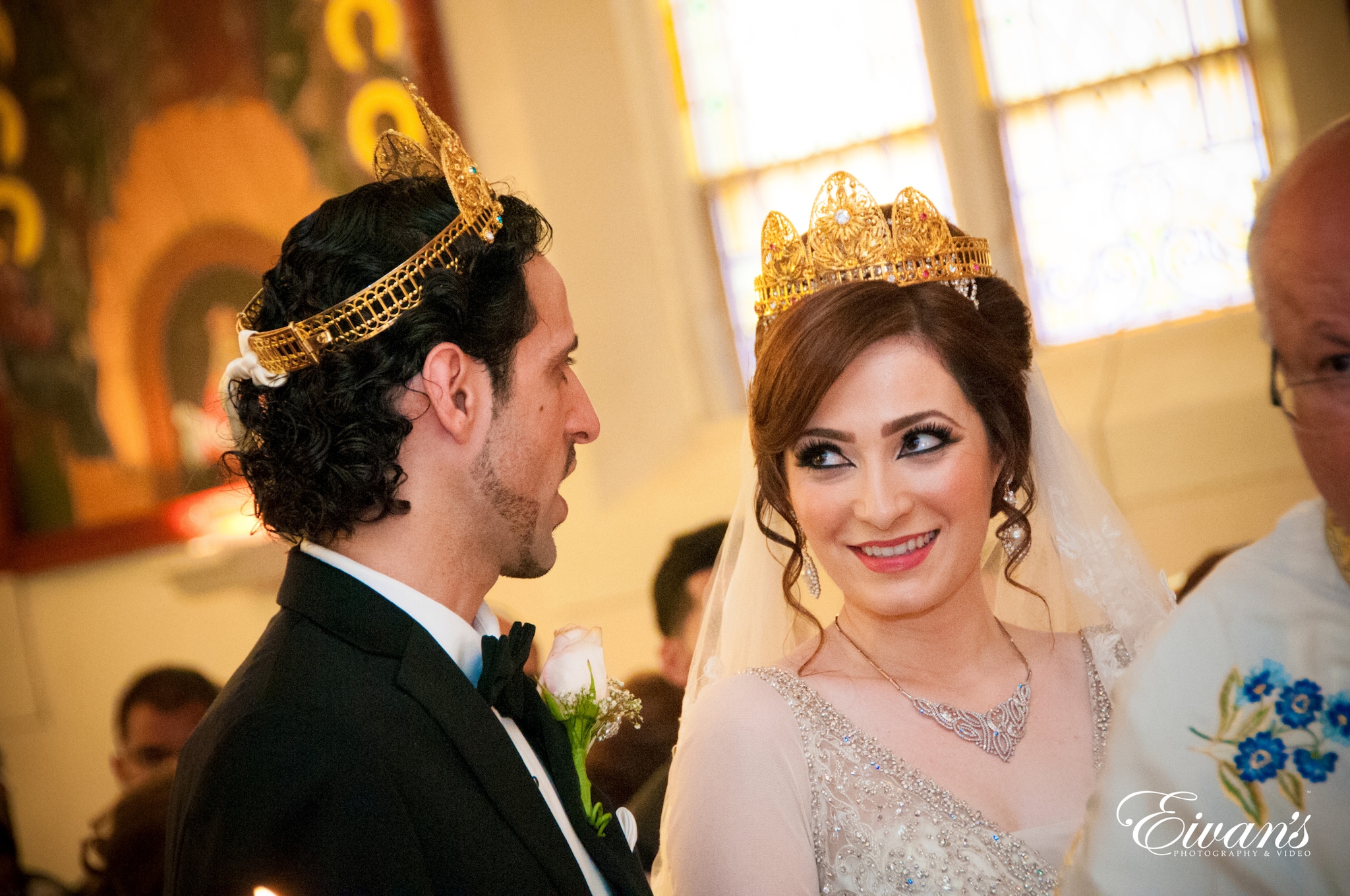This color photograph is a horizontal, landscape-oriented image capturing the joyful moment of a wedding ceremony in a church. At the center, the bride radiates with a bright smile as she looks lovingly at the groom. She has brown hair styled with tendrils and curls framing her face, adorned with a gold crown featuring three arches and a white veil cascading down the back. Her ensemble includes glittery gold and white gown, a large crystal pendant necklace, and drop earrings.

To the bride's left, the groom faces her, his mouth slightly open as if speaking to her, revealing his happiness. He wears a black tuxedo with a bow tie, a white shirt, a white corsage on his lapel, and a crown identical to the bride’s atop his short black curly hair. His dark eyes are fixed on her, adding to the intimate exchange between the couple.

On the right of the frame, partially visible, is a clergyman, presumably officiating the ceremony. He is depicted with a bald head and gray stubbly hair, thin-rimmed glasses, and a distinguished white robe decorated with blue flowers and gold leaves. The background of the image is slightly blurred but suggests the interiors of a church with large windows, a significant painting in the upper-left corner, and attendees seated in the pews.

In the bottom-right corner, the photographer's watermark "Eivans," stylized as E-I-V-A-N-S, is visible in white cursive text. The image is a detailed and representational capture of this sacred and celebratory moment.